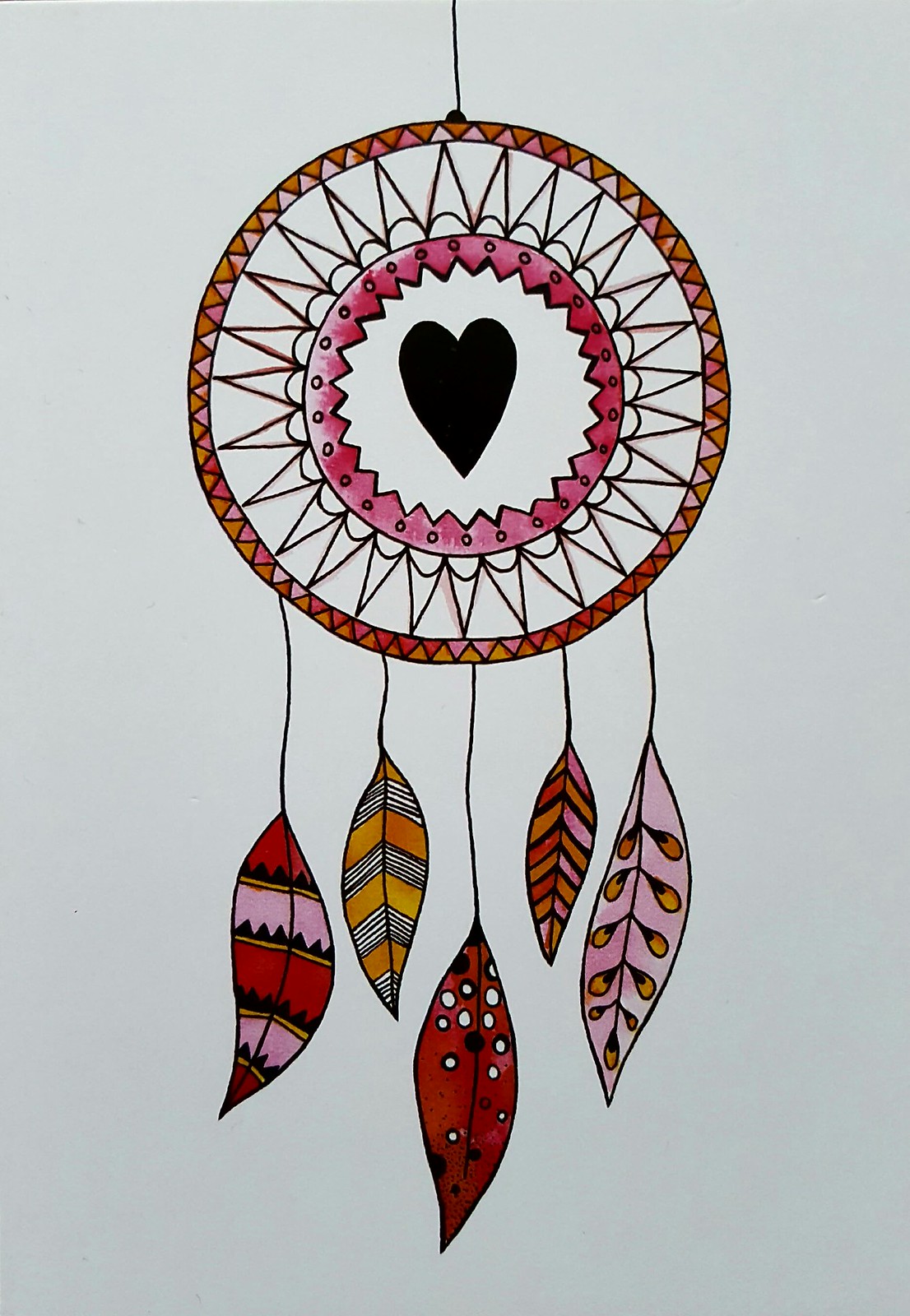This image features a detailed and colorful drawing of a Native American dreamcatcher, set against a pale gray background. It's suspended by a black string from the top. The dreamcatcher consists of two main circular sections. The outer circle is adorned with a crisscross pattern of orange, black, and white triangles. Within this, an inner circle hosts a red and white starlight pattern with distinctive rays shaped like little triangles. At the very center lies a solid black heart, cartoon-like in its simplicity, surrounded by a reddish ring patterned with white dots that match the triangle tines of the inner ring.

Hanging from the lower edge of the dreamcatcher are five artistic feather-like shapes, each uniquely colored and patterned. The first feather features shades of red, pink, and black. The second combines orange, black, red, and white with white dots. The fourth feather mixes pink with orange, while the fifth is primarily orange with pink seed-like designs extending from a central black line. This meticulously drawn dreamcatcher blends traditional cultural motifs with vibrant, modern artistic elements.